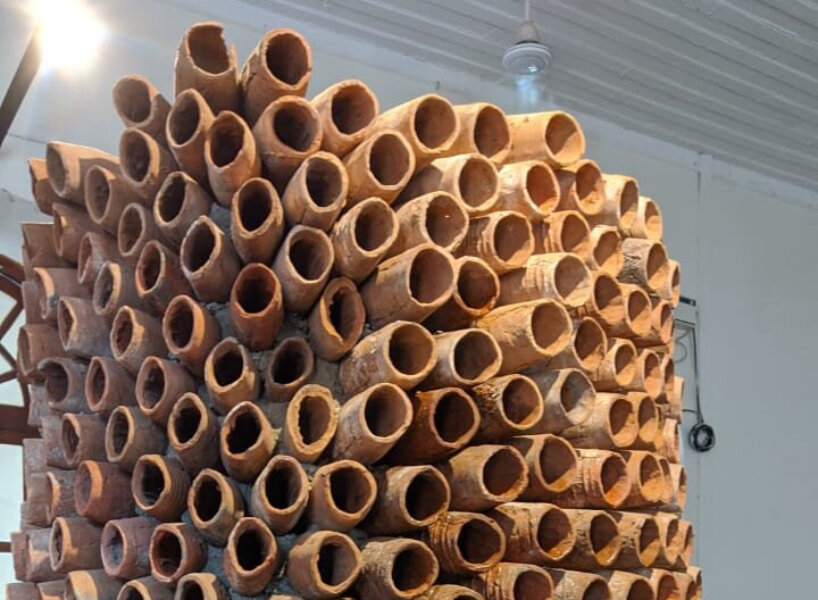The photograph depicts a rectangular, horizontal arrangement of what appear to be terracotta tubes stacked intricately on top of each other, resembling a hive. These tubes are embedded into a cement or mud-like substance, giving the impression of a cohesive and deliberate design rather than a construction material in storage. The setting appears to be an open space, possibly a warehouse or an area under a breezeway, characterized by white walls and rustic elements like a hanging Edison light bulb and another light in the upper left corner that illuminates the scene. Additionally, part of a wooden framework and what might be a window or doorway can be seen in the background, enhancing the industrial or modern art ambiance. The configuration of the tubes, with their round, cave-like entrances, looks too orderly for a natural hive, suggesting it might be an intricate piece of modern art. The photograph itself appears to be a casual snapshot rather than a professionally taken image, further emphasizing the raw and authentic feel of the scene.